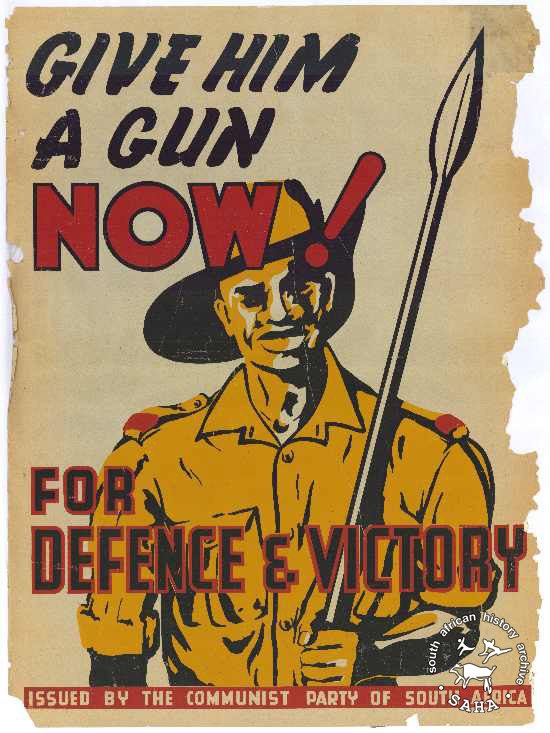This photograph showcases a vintage propaganda poster issued by the Communist Party of South Africa. The poster, now frayed at the edges and sporting a brown-yellowed tint, features bold and striking lettering in black and red, stating, "Give him a gun now!" and "For defense and victory." The central image depicts a stylized figure of a man, rendered in a warm color palette of yellows and reds, holding a spear. Though the man's features suggest he may be African, the artistic style does not use traditional black coloring. Notably, there is a watermark from the South African History Archive (S-A-H-A), indicating the poster's archival provenance.